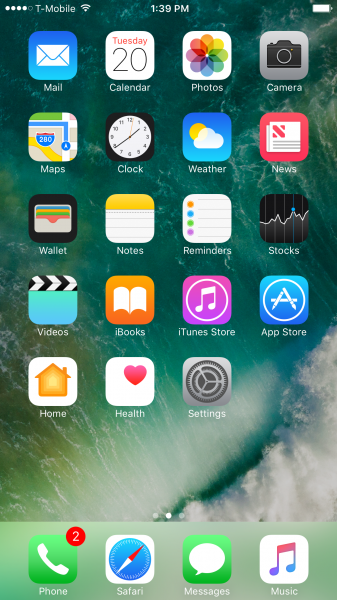The screenshot displays the home screen of an iPhone. In the top-left corner, the status bar indicates that four out of the five signal circles are lit, showing a strong connection to T-Mobile, and the Wi-Fi is enabled. The time displayed is 1:39 PM. In the top-right corner, the battery icon shows that the phone is nearly fully charged.

The home screen consists of five rows of app icons, with each row containing four apps:
- **Top row**: Mail, Calendar, Photos, Camera
- **Second row**: Maps, Clock, Weather, News
- **Third row**: Wallet, Notes, Reminders, Stocks
- **Fourth row**: Videos, iBooks, iTunes Store, App Store
- **Fifth row**: Home, Health, Settings

At the bottom of the screen, in the dock area, there are four apps: Phone (with two notifications), Safari, Messages, and iTunes (Apple Music).

The background image of the iPhone appears to be a natural scene, possibly depicting either a large waterfall or a close-up of a crashing wave. The image features white, frothy water prominently in the bottom right-hand corner, though the perspective makes it difficult to ascertain whether it is indeed a waterfall or a wave.